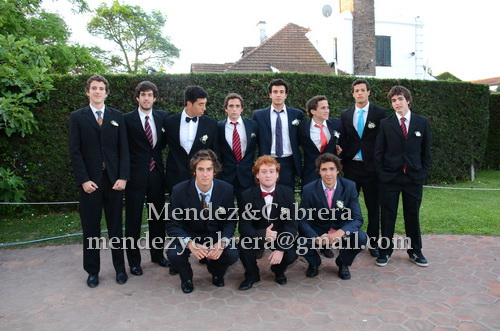The vibrant, sunny photograph captures a joyous moment of a graduation or fraternity celebration, taking place outdoors on a paved brick patio. The image features 11 young white men in their early to mid-20s, all smiling and dressed in black suits with white shirts. Their ties are a mix of styles, including several striped ties in red and blue hues, two bow ties, and a standout turquoise tie, with one individual opting for no tie at all. The men are arranged in two rows: eight standing in a straight line and three crouched in front. A tall hedge and a small grassy area serve as the backdrop, above which the rooftops and additional trees peek through, suggesting a backyard setting on a bright, midday. The professional touch is evidenced by the superimposed names "Mendez and Cabrera" along with their email address, likely indicating the photographers of this memorable occasion.